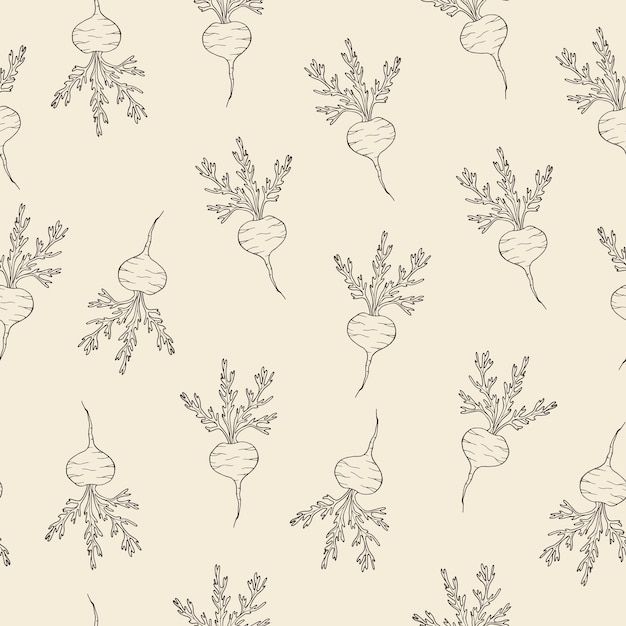The image displays a decorative pattern featuring hand-drawn illustrations resembling turnips, repeatedly outlined in black ink. These turnip illustrations cover a subtly hued background that is an almost eggshell beige color. Each turnip is characterized by a bulbous, chubby center with what appears to be tiger-like stripes on both sides, tapering down to a sharp, hair-thin point. At the top, they have leafy stems consisting of three to four leaves. Arranged in roughly six to seven diagonal rows, the turnips are angled at varying orientations, including right-side up and upside down, creating a balanced, evenly spaced design reminiscent of wallpaper.